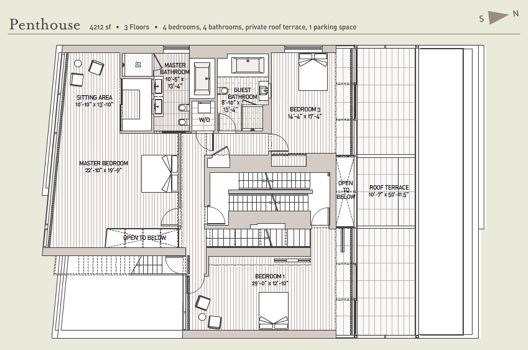This detailed floor plan image displays a luxurious three-story penthouse, Penthouse 4212, with a total area of 4,212 square feet. The layout includes four spacious bedrooms and four modern bathrooms. Highlighted features are:

- **Master Bedroom**: Positioned on the uppermost floor with an "open to below" area, providing an airy and elegant feel.
- **Private Roof Terrace**: Offering exclusive outdoor space for relaxation and entertainments.
- **Sitting Area**: Located on the top left corner, perfect for informal gatherings or serene reading sessions.
- **Guest Bathroom**: Conveniently situated for visitors' use.
- **Bedroom Layout**: Includes additional bedrooms thoughtfully distributed across the floors, ensuring ample personal space for all residents.
- **Parking Space**: Dedicated single parking slot.

Orientation is highlighted with a "South to North" marker in the top right corner, and the color scheme features a combination of brown and light green with a white space visible at the bottom left. The floor plan offers a comprehensive view of the penthouse's spatial distribution and upscale amenities.